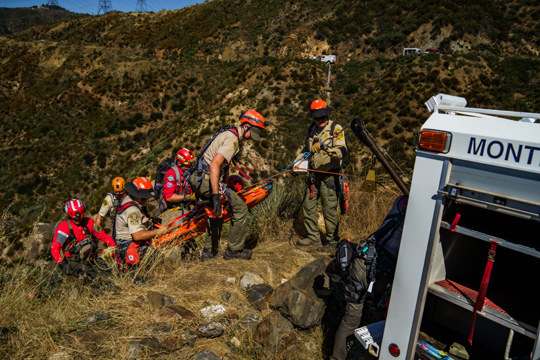The photograph captures a dramatic mountain rescue operation in progress. A group of first responders, clad in a mix of khaki shirts with green cargo pants and bright red high-visibility suits, diligently work to carry a stretcher up a rugged, bush-covered mountainside. Both groups are equipped with helmets—orange and red—often worn over baseball caps. The stretcher, a high-visibility orange type, partially obscures the individual being rescued, with only their head faintly visible.
   
The scene is set under a clear, bright blue sky, symbolizing a daytime operation. Towards the bottom right, a white emergency vehicle, possibly an ambulance, with the partially visible letters "M-O-N-T" and black straps hanging from it, sits with its back doors open. Adjacent to it are various pieces of equipment, mostly hidden from view, and a few other white vehicles are discernible in the background, enhancing the sense of urgency and coordinated efforts of the rescue team.